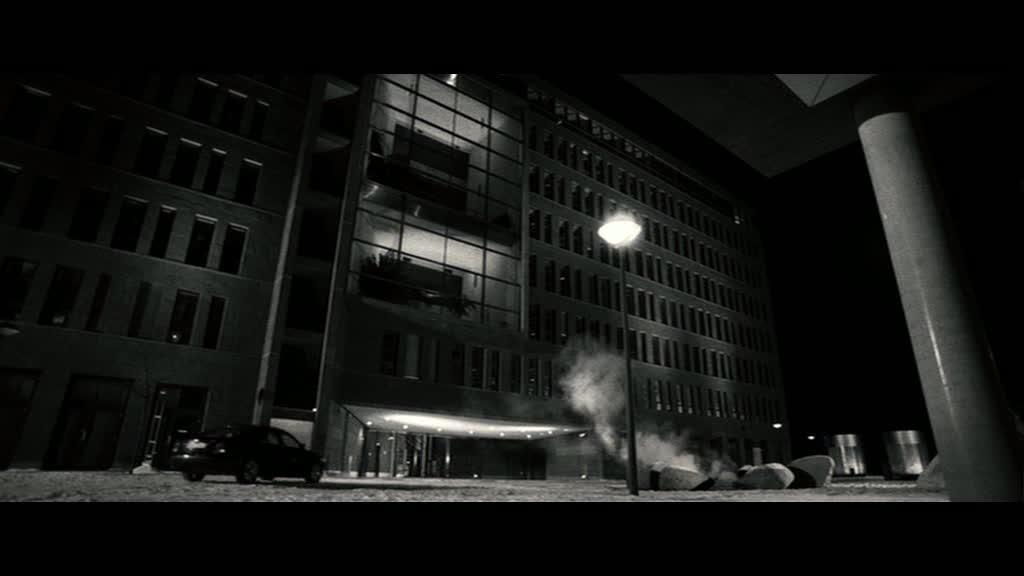This black and white nighttime photograph captures an eight-story office building with prominently visible doors at the ground level and large windows lighting up the facade. The building features a shiny, marble-like column to its left and a tall street lamp with a dark pole and light above. In front of the building, there is a black sedan parked to the left, though details of the car are obscured due to the dark setting. Smoke billows from beneath a vent near the building, suggesting an underground subway or some other source below the ground. Despite the windows being a significant feature, there appears to be no lights on within the building’s interior, adding to the image's mysterious atmosphere. The overall scene includes elements like additional cars passing by and further invokes a quiet, yet bustling urban environment at night.